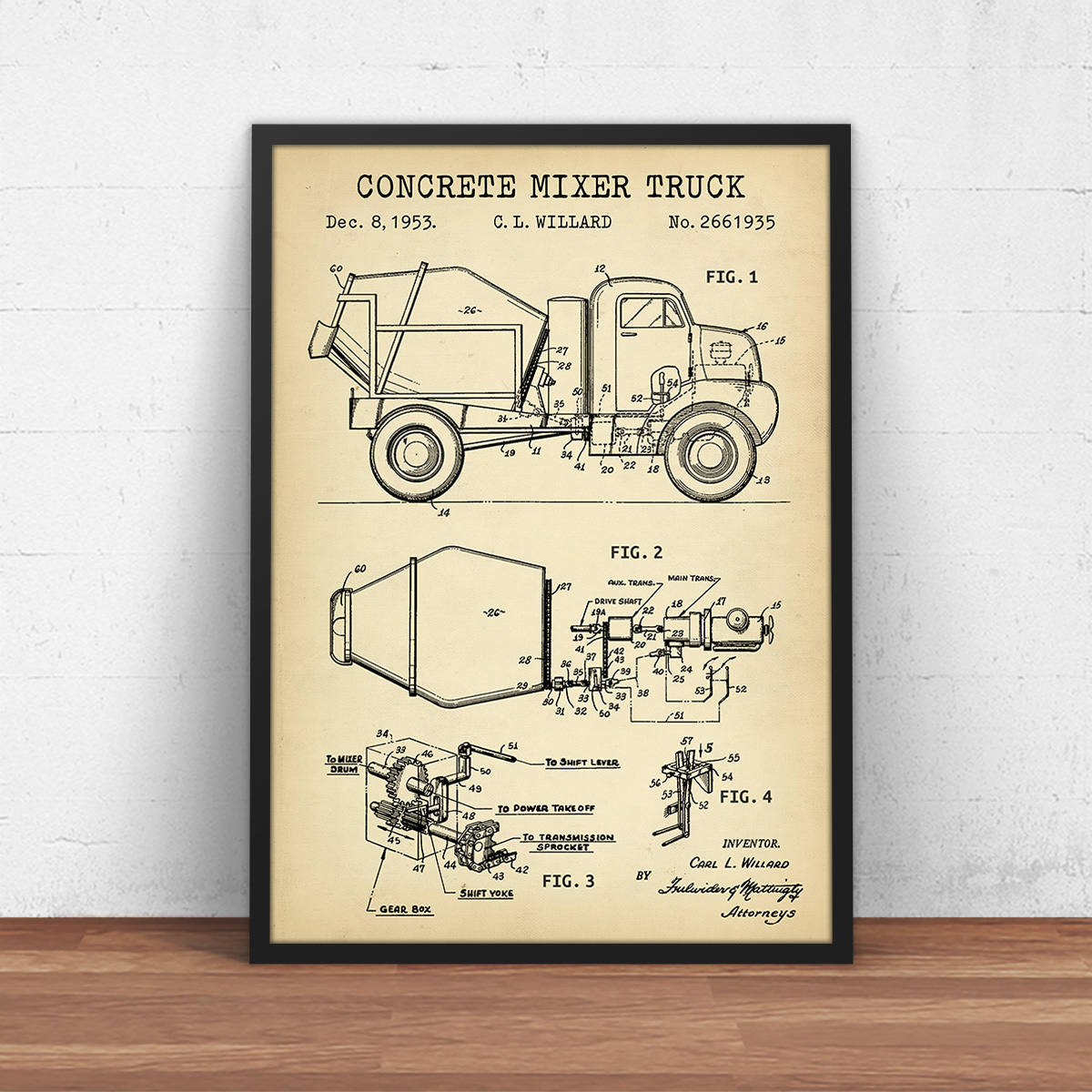The image captures a detailed, black-and-white line drawing framed in black and propped against a white, cinder block wall on a wooden floor. The drawing, titled "Concrete Mixer Truck, December 8, 1953, C.L. Willard, number 2661935," resembles a patent illustration, showcasing various labeled views and technical details of a concrete mixer truck. Figure one presents a side profile of the truck, figure two offers a top-down perspective of the mixer, figure three appears to illustrate internal gears, and figure four includes a smaller, indistinct part of the truck. The aged cream background of the drawing and the detailed labeling accentuate its technical, historical essence. The bottom section notes the inventor as C.L. Willard, along with mentions of attorneys, confirming its status as a patent document.